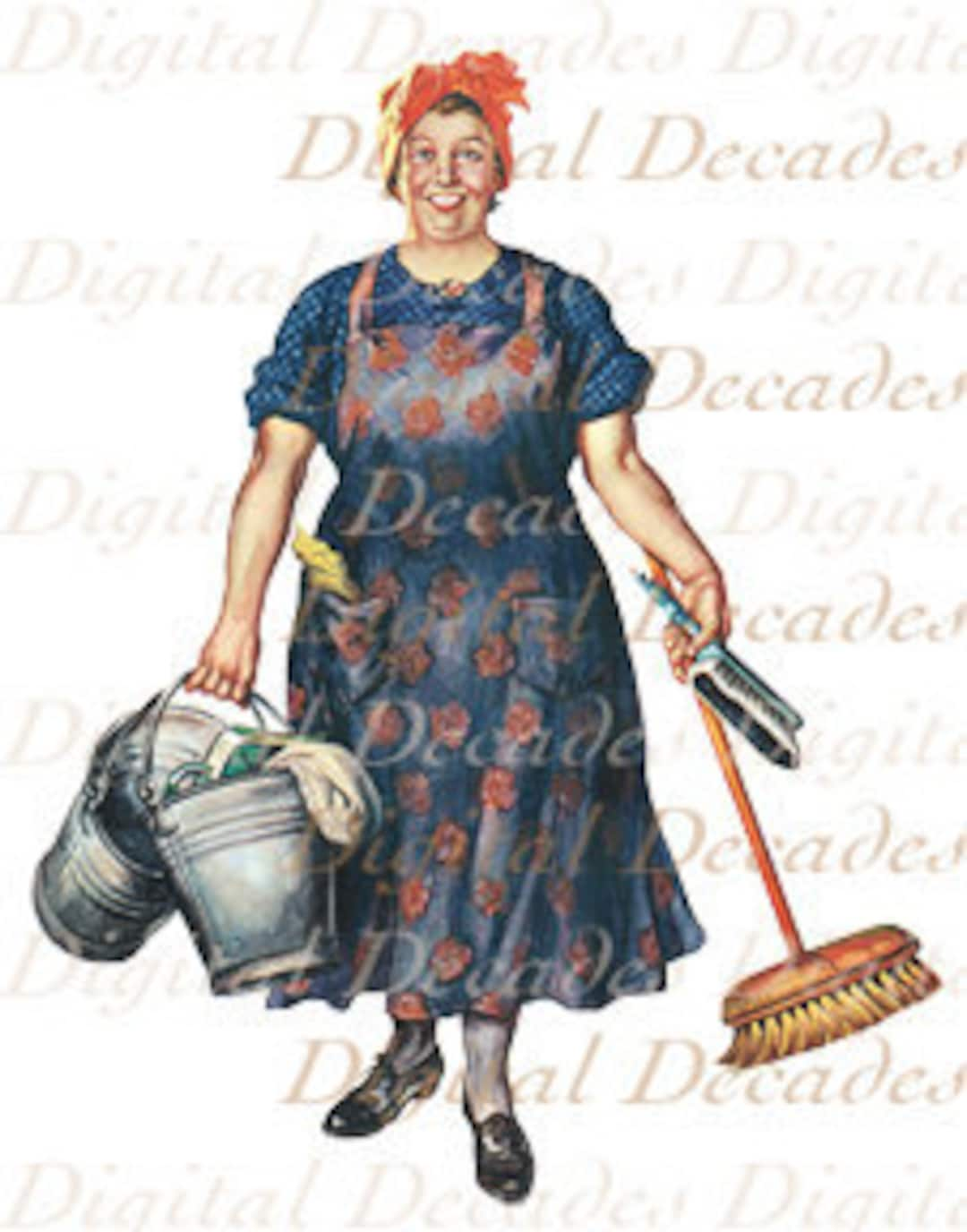The image showcases a cheerful, light-skinned, heavyset cleaning woman with reddish cheeks, smiling broadly. She is wearing a blue dress adorned with white dots and a red rose print apron. A yellow cloth peeks out from a pocket on her apron. Her head is wrapped in a pink handkerchief. In her left arm, which is awkwardly bent, she holds a broom and a bristle brush, while her right hand carries two metal buckets, with rags partially overflowing from them. She completes her outfit with white socks and shiny black shoes. The background features the words "digital decades" repeatedly in light brown script, adding a distinct watermark effect to the image.